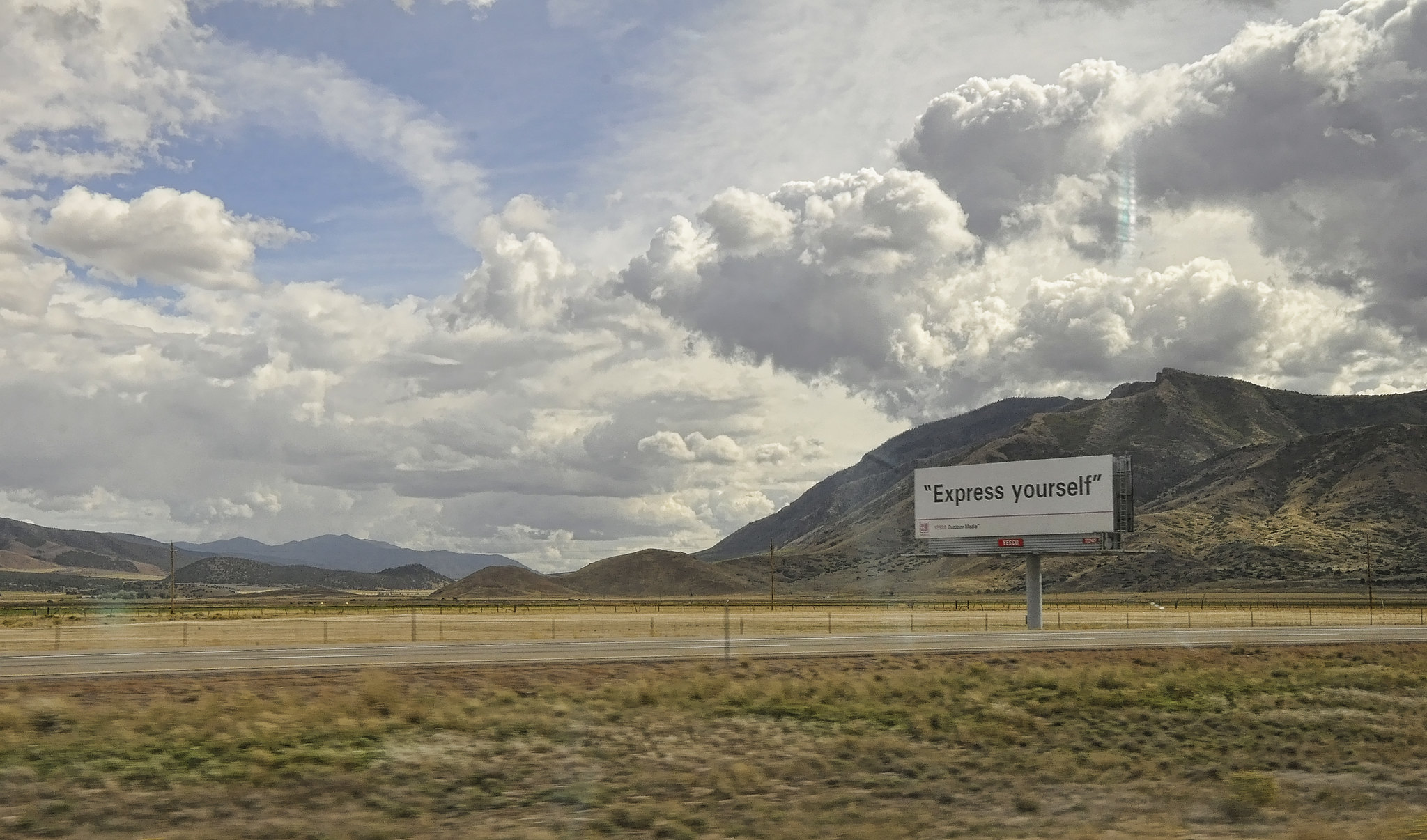This daytime photograph captures a varied scene of both natural and man-made elements. In the foreground, a patchy expanse of grass is visible, showcasing a spectrum of colors from light green to dark green interspersed with brown areas, alongside large clumps of exposed dirt. Stretching beyond the grass is a roadway, faintly marked with white lines. Dominating the middle of the image is a towering billboard mounted on a sturdy metal post. The billboard features a white background with dark font that reads "Express Yourself." In the background, a mountain-like formation is visible, its surface dotted with patchy green grass. Above, the sky is partially obscured by thick cloud cover, with one side appearing gray and the other transitioning to a lighter white, contrasting against patches of blue sky.